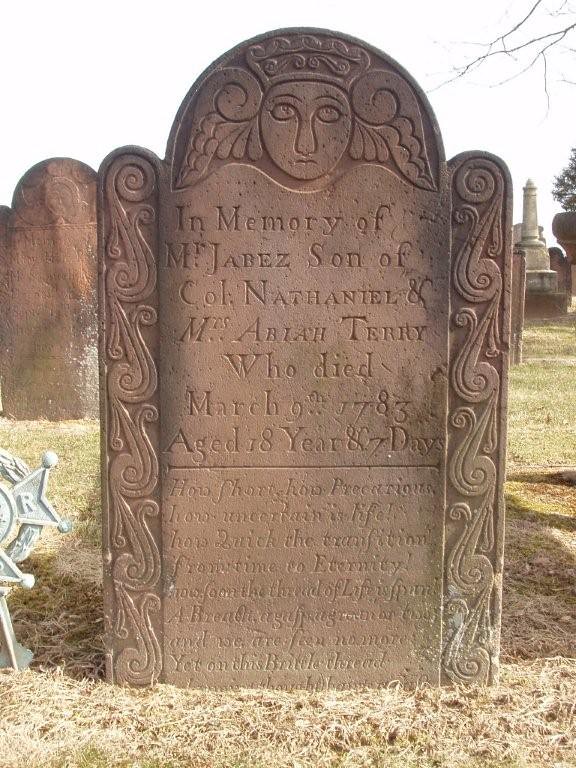This photograph showcases an aged tombstone with an arched top, predominantly light brown in color, transitioning to a beige hue near the bottom due to discoloration. The top of the tombstone features a stylized engraving of an angel with a crown, flanked by wings on both sides. The sides of the tombstone are adorned with a symmetrical, flourished design. Etched below the angel, the inscription reads: "In memory of M. Jabez, son of Colonel Nathaniel and Mrs. Abia Terry, who died March 9, 1783, aged 18 years and 7 days." Beneath this primary inscription lies a smaller, more difficult-to-read text imparting a poignant message about the brevity and uncertainty of life. The tombstone is situated amidst dried-up brown grass, emphasizing its weathered and time-worn condition.